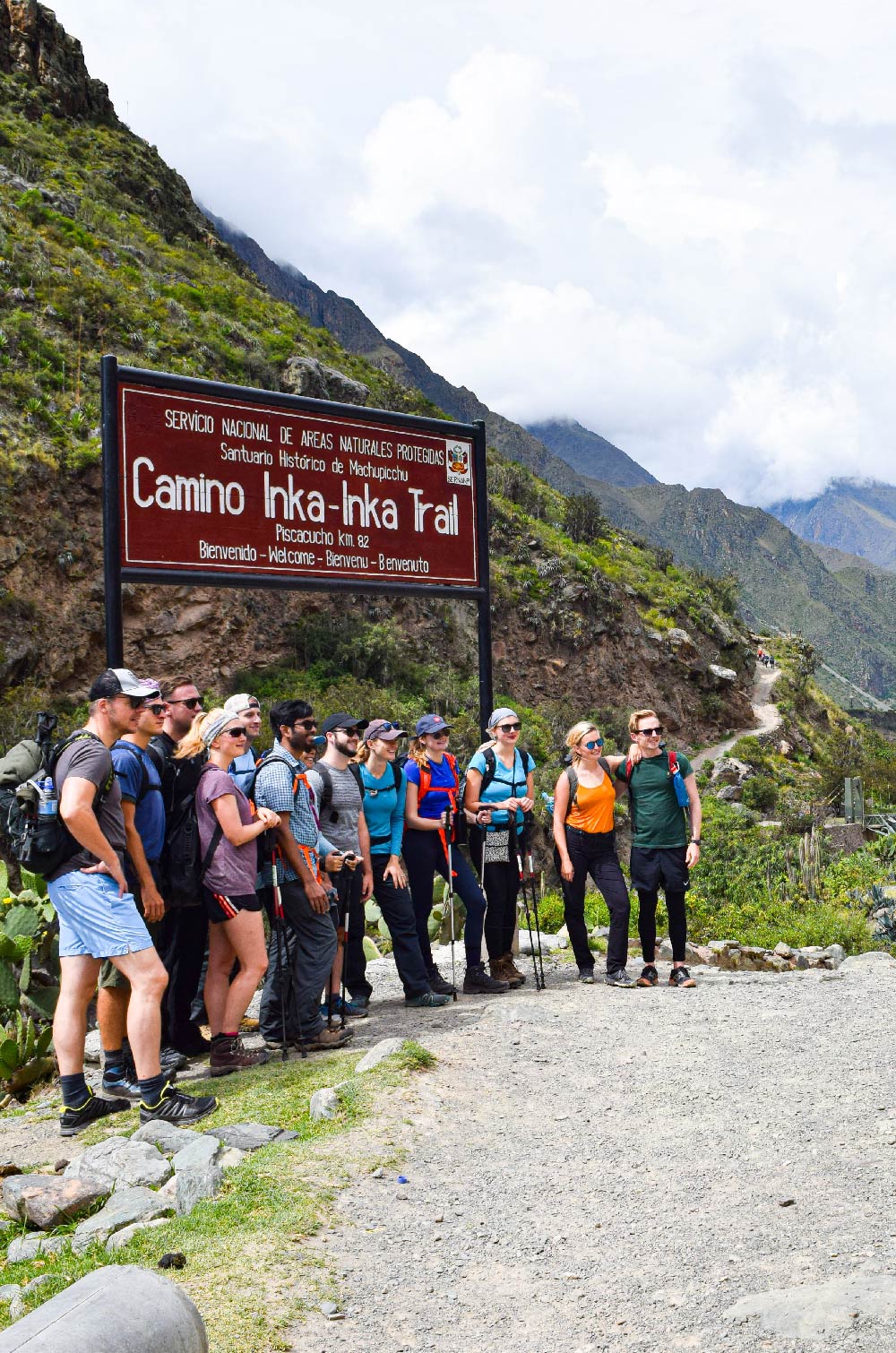In this color photograph, a group of approximately 12 hikers, both male and female, are gathered underneath a prominent red sign that reads "Camino Inca - Inca Trail" with additional Spanish text positioned above and below the primary inscription. These tourists, who appear to be taking a group photo, are equipped with various hiking gear, including backpacks and black walking sticks. They are dressed in a mix of hiking pants and shorts, capturing the spirit of adventure. The hikers are standing on a rocky, gravel-lined path, dotted with pebbles and larger stones. Their smiling faces are framed by the stunning backdrop of a mountainous landscape, partially shrouded in white clouds. The lush green mountains, devoid of trees but rich in grass and plant material, stretch into the distance, offering a vibrant contrast to the earthy foreground. The scene exudes a sense of camaraderie and exploration amidst the natural beauty of what appears to be a national park or well-trafficked hiking area.